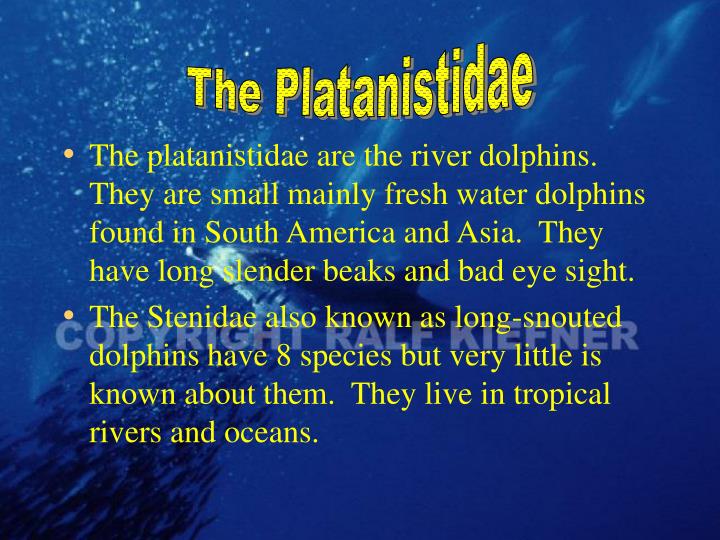The PowerPoint presentation slide depicts the Platanistidae family, commonly known as river dolphins. The background features an underwater scene with a blue ocean color, partially obscured images of a dolphin, some bubbles, and possibly small fish and a diver in the lower left. In yellow text, two bullet points describe these dolphins: first, they are small, primarily freshwater creatures found in South America and Asia, characterized by long, slender beaks and poor eyesight. Second, they are also known as long-snouted dolphins or the Stenidae family. There are eight known species, but little information is available about them. They inhabit tropical rivers and oceans. The slide is credited to Ralph Kiefner.